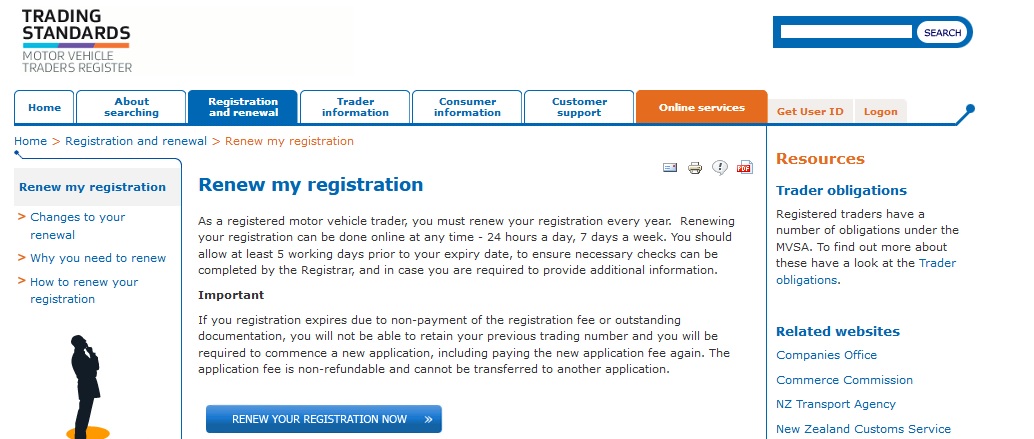The image displays a website interface with a header titled "Trading Standards" located in the top-left corner. Below the header is a colorful banner featuring teal, purple, and orange accents that reads "Motor Vehicle Traders Register." On the extreme right side of the header, a search bar is accompanied by a white button labeled "Search" in black text.

Below the header, a horizontal menu bar contains several navigational tabs:
- "Home" (white background)
- "About Searching" (white background)
- "Registration and Renewal" (highlighted in blue indicating the current section)
- "Trader Information" (white background)
- "Consumer Information" (white background)
- "Customer Support" (white background)

To the right of the menu tabs, there are three buttons:
- An orange button labeled "Online Services"
- A gray button with orange text that reads "Get User ID"
- Another gray button similarly labeled "Login" with orange text

In the main content area, near the bottom, there are several paragraphs of text that provide information about renewing registrations. A clickable link at the bottom of this section prompts users with the message, "Renew your registration now."